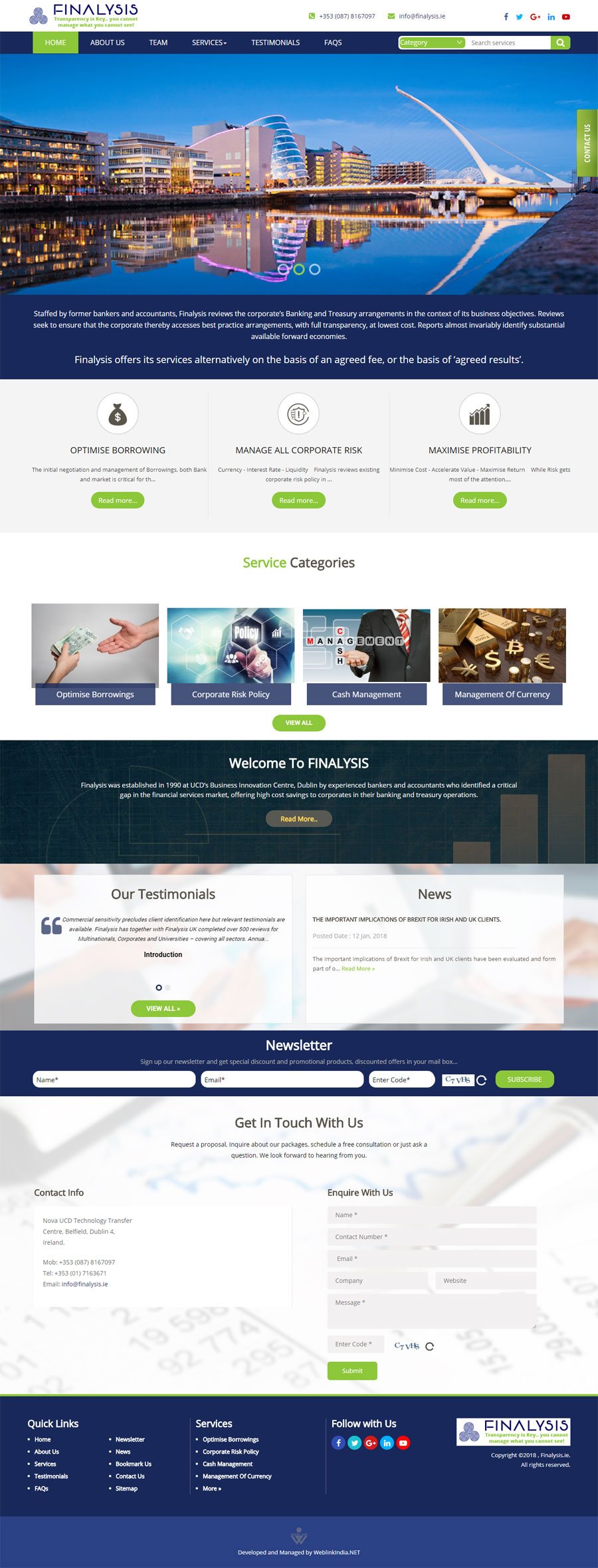This image is a detailed view of the homepage of Vanalysis, a Dublin-based corporate banking and treasury consultancy established in 1990 by former bankers and accountants. The company’s name is uniquely stylized, with the 'A' depicted as an upside-down 'V,' emphasizing their philosophy that "Transparency is key; you cannot manage what you cannot see." 

Prominent contact options include their phone number, +353 07 816 7097, adjacent to a small green phone icon, and their email address, info@vanalysis.ie. Additionally, their social media links for Facebook, Twitter, Google Plus, Instagram, and YouTube are provided for further engagement. 

The website has a navigation bar with a green-highlighted 'Home' button, and options to learn more about the 'About Us,' 'Team,' 'Services,' 'Testimonials,' 'FAQs,' and a category search for services. 

A captivating background image showcases a beautiful outdoor scene under a vivid blue sky, featuring tall buildings – possibly hotel resorts or corporate offices – overlooking a serene lake or pool. The scene appears to be captured in mid-evening, as building lights are on, complementing the tranquil atmosphere depicted. 

The homepage content describes Vanalysis’s objective to review corporate banking and treasury arrangements, aligning them with business goals. They offer services on either an agreed fee basis or based on achieved results, optimizing borrowing, managing corporate risk, and maximizing profitability. 

Four distinct images illustrate their services: one shows a person handing money with two hands, representing financial transactions; another depicts a corporate risk policy with a central hand gesture indicating a 'no' from a man in a suit with a red and white tie; the third image shows cash management; and the fourth highlights currency management with gold coins representing various currencies.

The text welcomes visitors to Vanalysis, celebrating its longevity and expertise. The website also features sections for testimonials, news, and quick links to their services, all against a cohesive and visually pleasing design, with a blue background at the footer enhancing the professional feel.